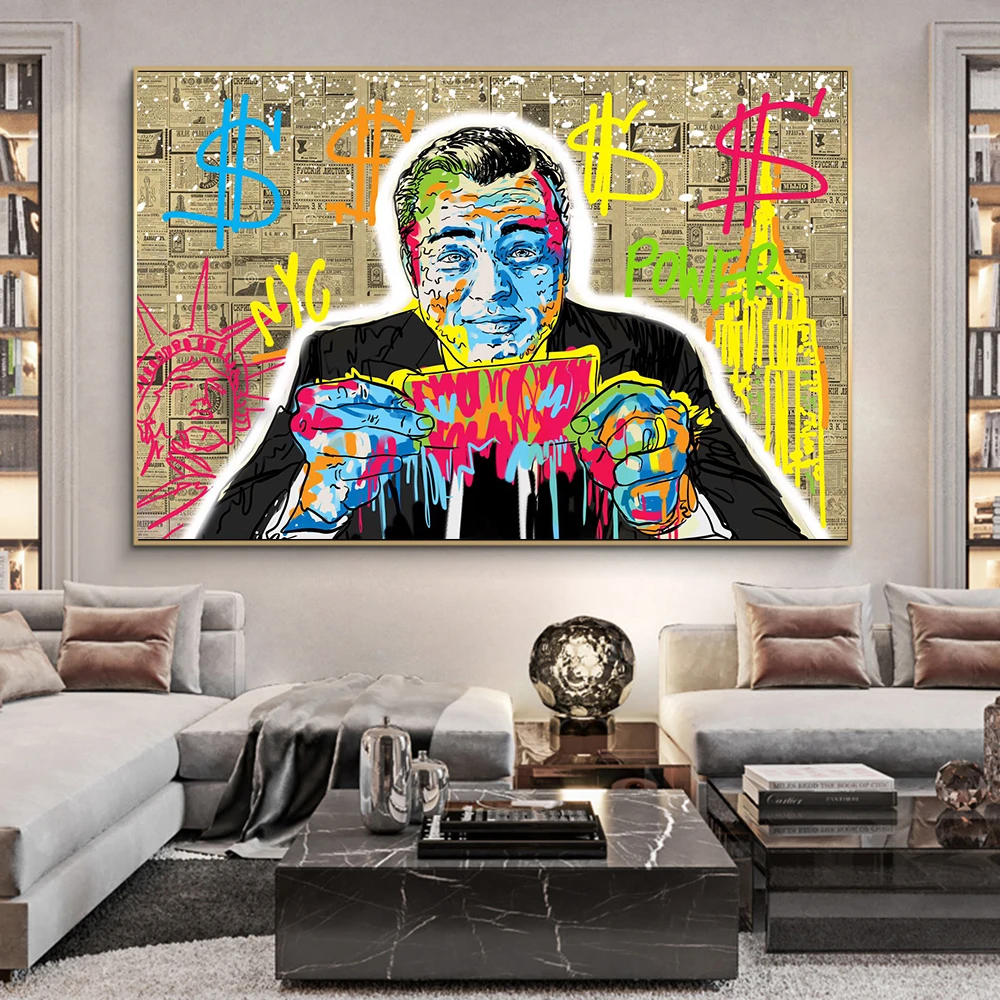The image showcases an indoor space, possibly a living room or a large seating area in an apartment or hotel. The room features multiple grayish couches adorned with brown pillows. Situated in front of these couches is a black coffee table cluttered with books and artistic objects, including what appears to be silver flasks. Mounted prominently on the wall behind the couches is a large, vibrant piece of artwork. This artwork depicts a man who bears a resemblance to Leonardo DiCaprio, dressed in a black jacket. His face and hands are adorned with bold, multicolored splotches of blue, red, yellow, and green. He is holding a piece of paper, resembling a dollar bill, which is also colored with various hues. The background of the artwork consists of newspaper clippings, and crudely drawn dollar signs, alongside depictions of the Statue of Liberty and the Empire State Building. Text in the background reads "NYC" in yellow and "Power" in green, positioned on the left and right sides of the figure respectively. Additional bookshelves flank the area, adding to the intellectual ambiance of the room.